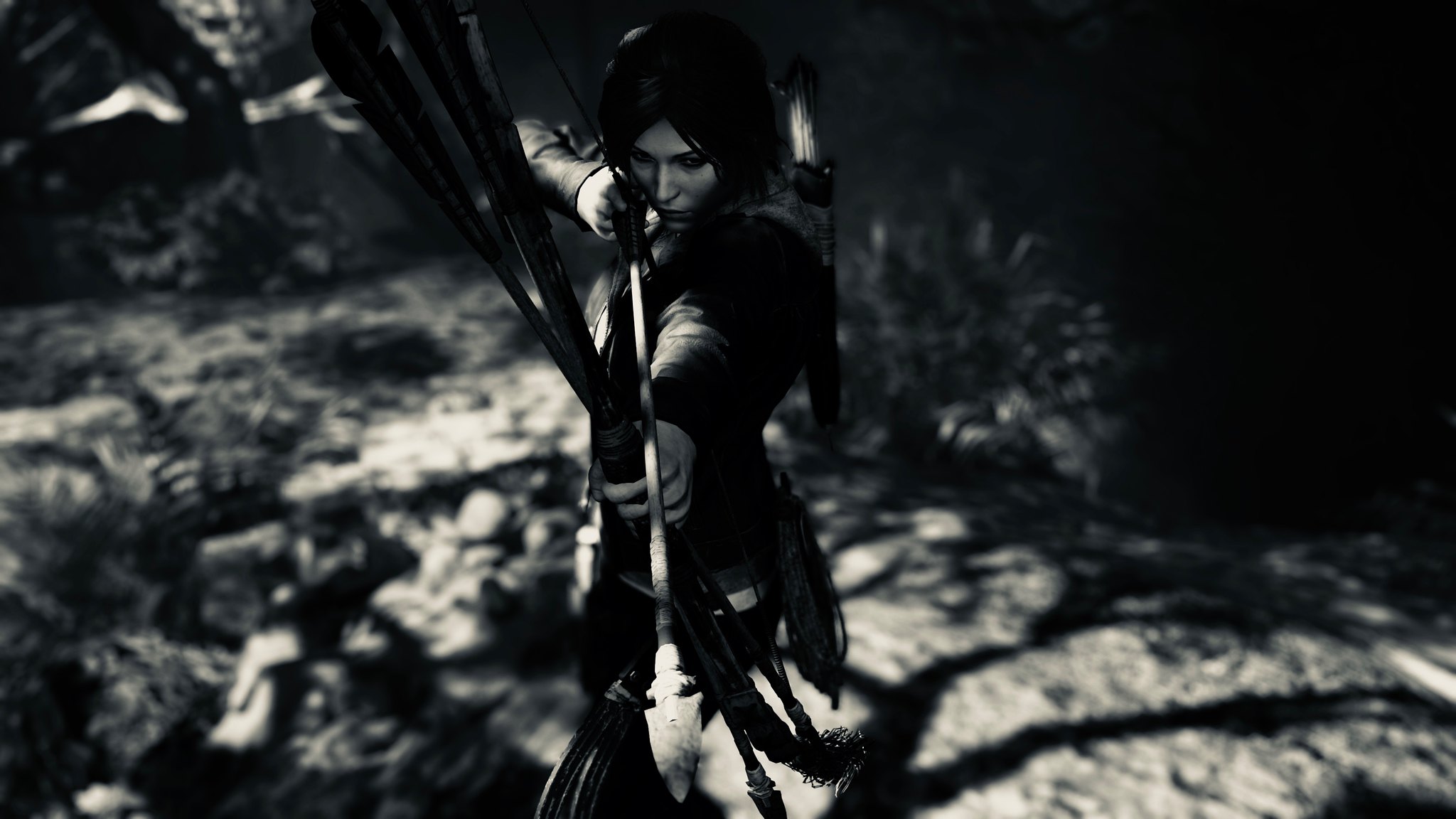A black and white screenshot from a modern, high-end video game shows a computer-generated image of a woman in a wooded area, potentially hunting. Viewed from a slightly elevated, top-down perspective, the woman appears to be in her 20s or 30s with medium, shoulder-length hair. She stands in a forest, drawing back an arrow on a large bow with her right arm, aiming at a target below the camera's view. The details in the image, such as the shadows of trees on the ground, shrubbery, and other environmental aspects, suggest a lush, forested setting. The arrow in her bow seems to have a flint head, hinting at a fantasy theme. This meticulously captured image underscores the intricate graphics and immersive nature of the game.